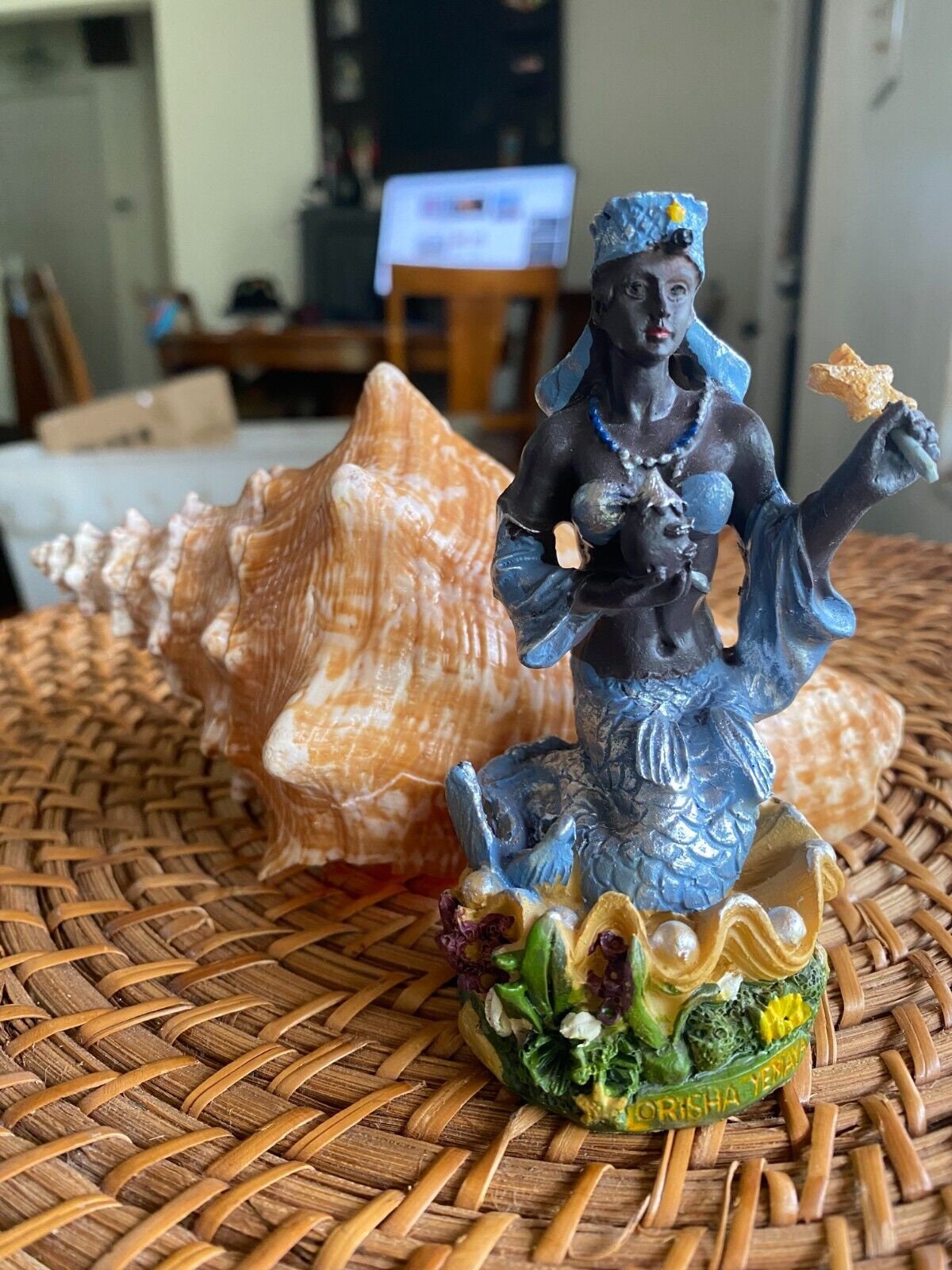The photograph showcases a detailed indoor scene centered around a white table adorned with a round, woven mat. On this mat sits an ornate statue of a mermaid, who is depicted in a seated position within a large, orange-yellow oyster shell accented with white highlights. The mermaid, identifiable as Yamaya, from the inscription "Orisha, Yamaya" on the sculpture, holds a starfish in her left hand and is dressed in a blue bikini top and blue fins that extend from her waist down. She has decorative sleeves on her arms, also blue, and wears a flat hat on her head. Additionally, pearls can be seen around the shell, enhancing the seaside theme of the decoration. In the background, there is a chair positioned at an office desk with a lit computer screen and a flat-screen TV mounted on the gray wall above the desk. A box is also visible on the table in the far background, contributing to the detailed setup of the room.